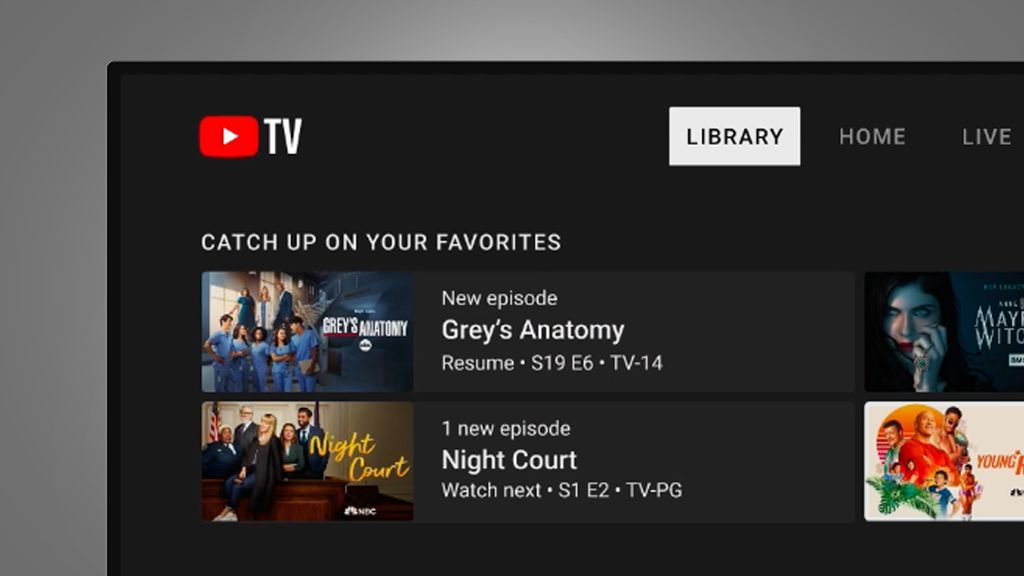This image depicts a television screen featuring a streaming service interface. The majority of the screen’s content is visible, though parts are cut off, predominantly towards a solid gray background. The top section shows several navigation icons: "TV," a play symbol, "Library," "Home," and "Live," with "Library" highlighted within a white box and black letters.

Beneath this navigation bar, the text "Catch Up on Your Favorites" is prominently displayed on the left. Below this, there is a promotional tile for "Grey's Anatomy," a popular ABC series about doctors. The image within the tile shows a group of doctors in scrubs standing on a stairway. Information displayed includes "New Episodes," "Grey's Anatomy," and an option to "Resume" watching from "Season 19, Episode 6," rated TV-14.

Directly below this, there is another tile for "Night Court," indicating a new episode available to watch. It prompts the viewer to watch the next installment, which is "Season 1, Episode 2," rated TV-PG. The image shows several people in a courtroom setting, either sitting or standing, with an American flag visible in the background.

To the right, two more tiles are partially visible. One shows "The Young Rock,” while the other appears to be a show featuring witches but is cut off, leaving the title unclear.